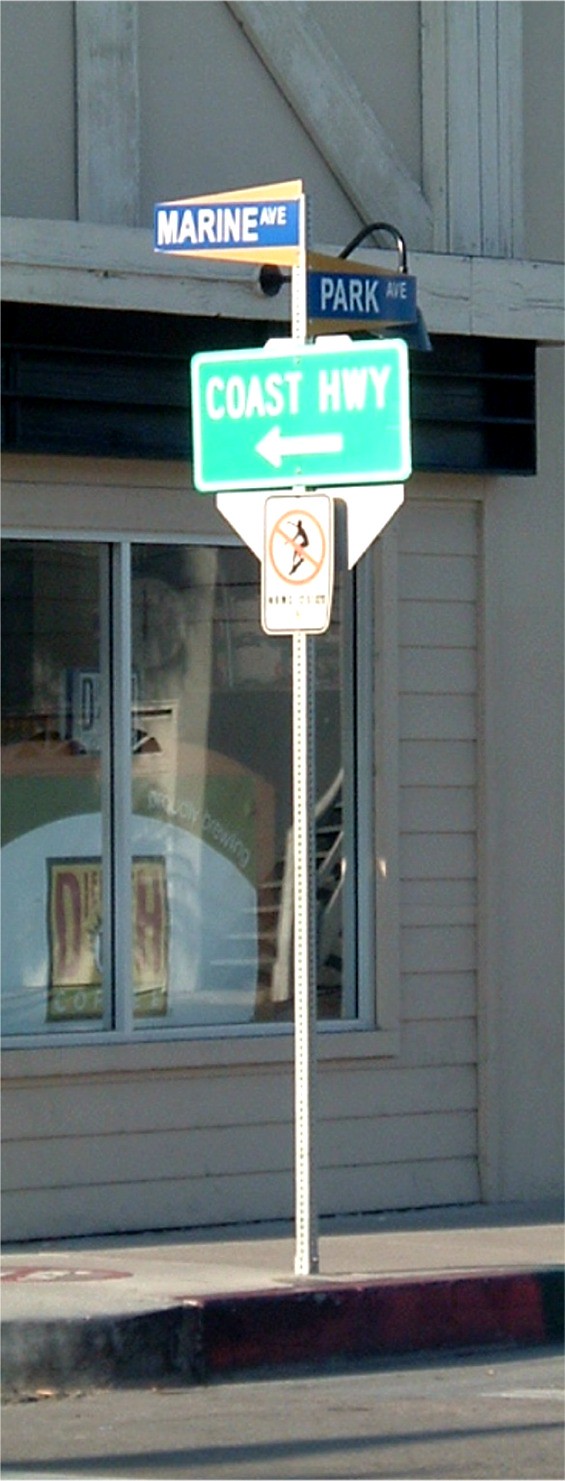The image depicts a street scene dominated by road signs and a cream-colored building with siding. The prominent street pole, embedded in a gray sidewalk elevated slightly above the street, holds multiple signs. At the top, two blue rectangular street signs indicate Marine Avenue and Park Avenue in different directions. Directly below, a green horizontal sign reads "Coast Highway" with an arrow pointing left. Beneath this is a red circular sign featuring a crossed-out silhouette of a surfer, implying no surfing.

Against the background, the building features a large window with a thin metal partition. Inside, partially visible is a white sign with green trim, with the word "coffee" clearly displayed at the bottom. Additional details include a white clock with black numbers hanging on the wall inside the building. The sunny outdoor setting casts long shadows, indicating the sun is positioned low in the sky.